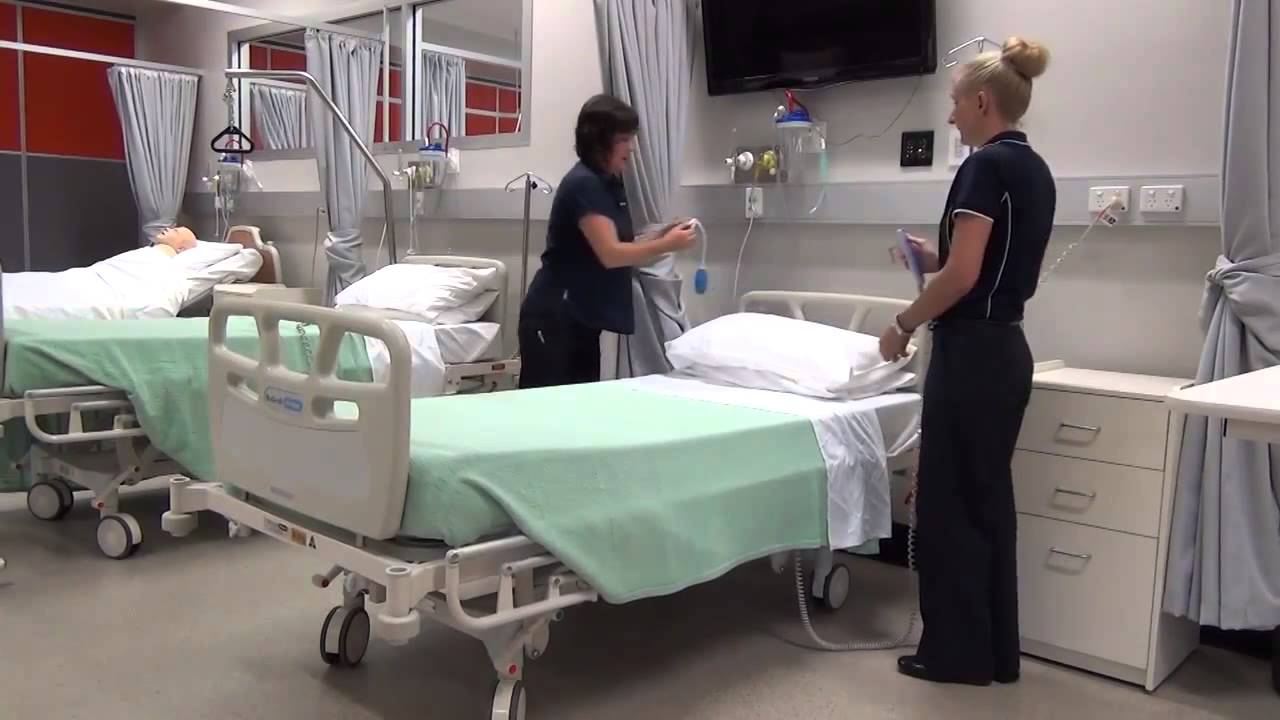The image shows a hospital room with three beds, each equipped with wheels and covered in green sheets complemented by white pillows. One bed in the back has a patient, a white male, while the two beds in the foreground are empty. Two women, likely nurses or doctors, stand on either side of the nearest bed, which features an attached little drawer. They are dressed in black or navy blue outfits and are holding objects that appear to be cables or gadgets meant to attach to the wall, possibly for setting up or calibrating the bed. The room's floor is tan brown, and the walls are white, adorned with a flat-screen TV.